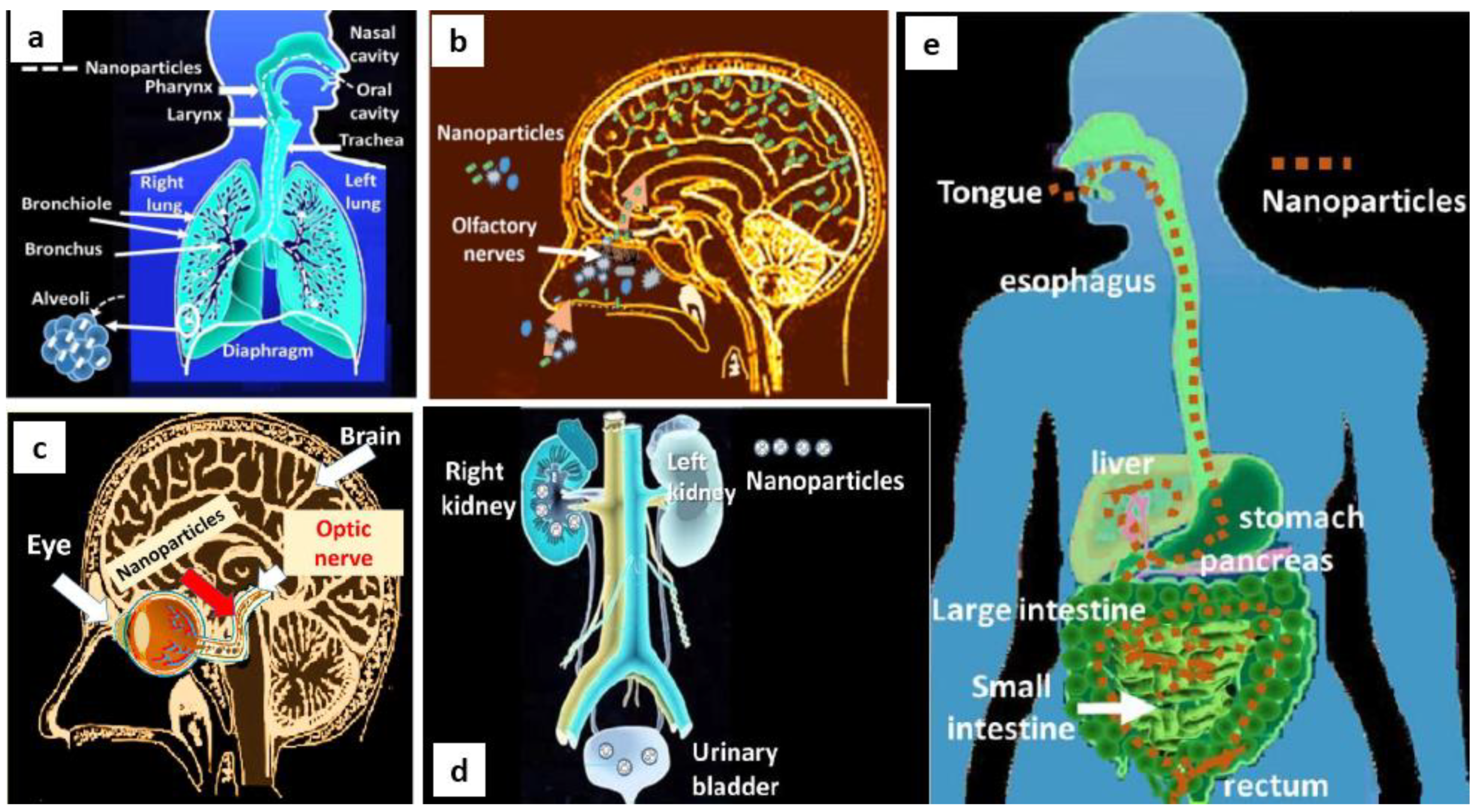The image presented consists of five detailed diagrams illustrating various human anatomical systems, each marked with a label from A to E. To the left is a quadrant arrangement of four square sections, and to the far right is a vertically oriented rectangle.

- **Image A** in the top left corner depicts a detailed diagram of the respiratory system, including the nasal cavity, trachea, bronchioles, bronchus, alveoli, pharynx, and larynx, all intricately labeled. The background is black, and the anatomical structures are highlighted in a bluish outline with white text and arrows pointing to each part.

- **Image B**, located to the right of the first image, focuses on the human brain. Set against a brownish-reddish backdrop, this diagram details the cranium, olfactory nerves, and various regions of the brain, all marked with white arrows and text.

- **Image C**, situated in the bottom left, presents an image of the human eye and sections of the brain, emphasizing the optic nerve. The background remains black, featuring a bluish outline of the structures and white labeling for clarity.

- **Image D**, directly to the right of Image C, illustrates the urinary system, showing both the left and right kidneys, along with the urinary bladder. This image uses a combination of blue and tan colors to differentiate the arteries, complemented by white text annotations.

- **Image E**, the vertical rectangle on the far right, displays a comprehensive view of the digestive system from the tongue down to the rectum. This includes the esophagus, liver, stomach, pancreas, large and small intestines, all outlined in various colors with white text and arrows for easy identification.

In all diagrams, the term "nanoparticles" appears prominently, linking the images to the study of how these particles interact with different bodily systems. The consistent use of a black background and white labeling, combined with colored anatomical outlines, provides a cohesive and clear presentation intended for detailed medical or scientific analysis.